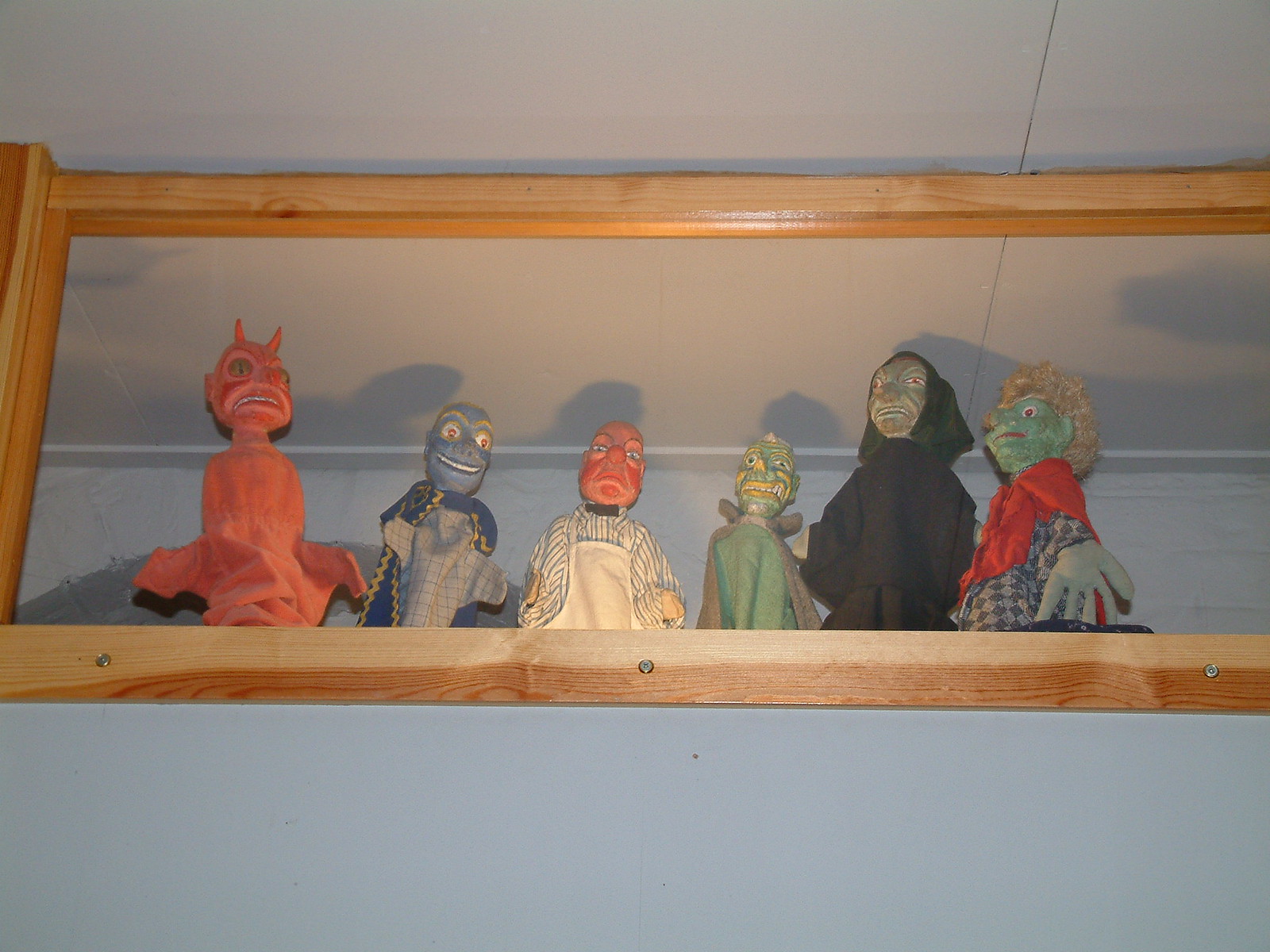The photograph captures a group of six puppets arranged in a recessed, framed display on a wall within a room with low lighting. The puppets, which likely have cloth bodies and painted wooden heads, exhibit a variety of eerie and monstrous characteristics. Each puppet is distinctive in appearance:

1. The leftmost puppet is a red devil with horns and a frowning or grimacing expression.
2. Next to the devil is a blue puppet with large, wide eyes and a smile, featuring some gold accents.
3. The third puppet resembles a butcher or chef, with a red face, a white apron, and a striped shirt.
4. Fourth in line is a green zombie-like figure with a snarling expression.
5. The fifth puppet, donning a black hood and robe, has a sinister demeanor reminiscent of a Grim Reaper.
6. The final puppet on the right is green, with curly hair, a red shirt, and blue-checkered pants.

All these puppets are set against a light blue-grey wall, framed by a wood structure that appears tan-orange and is held up by screws. This display shelf is mounted high on the wall, and the photograph is taken from a slightly lower angle, enhancing the creepy atmosphere. The ceiling tiles visible in the background are white, adding to the overall eerie ambiance of the scene.